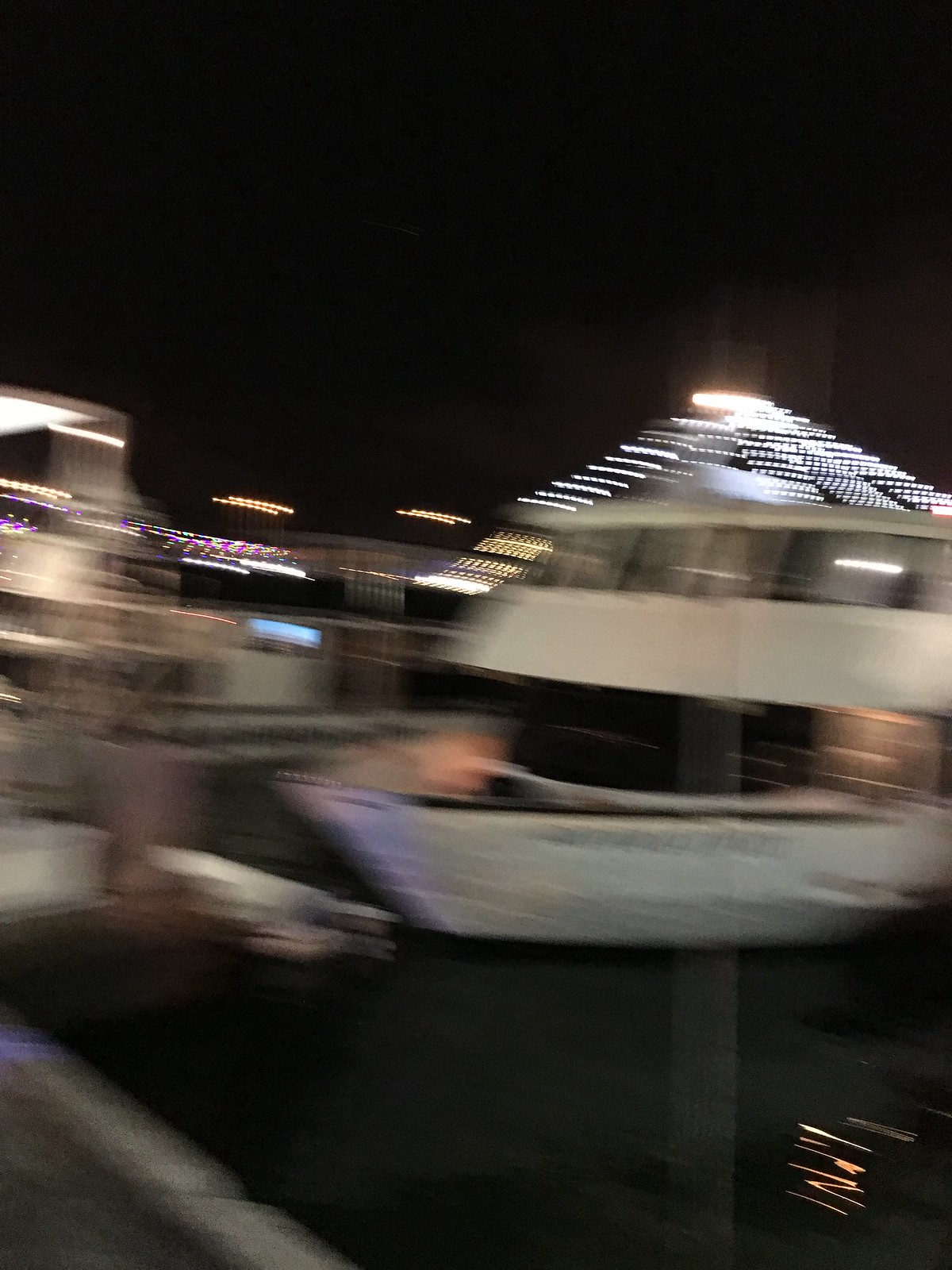In this photograph, the scene is enveloped in a very dark background, creating an overall dim and moody atmosphere. The image itself is significantly out of focus and extremely blurred, making the details hard to discern with precision. Across the upper portion of the image, there appears to be a horizontal demarcation which likely represents a concrete wall, framing a body of water below. 

Dominating the scene is a large, white, two-story boat positioned near the water's edge. This vessel features a dark roof, several windows, and seats visible through the blur. Atop the boat, a light fixture is faintly discernible. Down in the lower right corner of the picture, there is a small, indistinct scribble in a pinkish hue that stands out against the darkness, though its significance is unclear.

In the blurry background, the faint silhouettes of additional boats can be seen, blending into the obscurity of the scene. The combination of the dark, unfocused elements gives the image a somewhat mysterious and impressionistic quality.